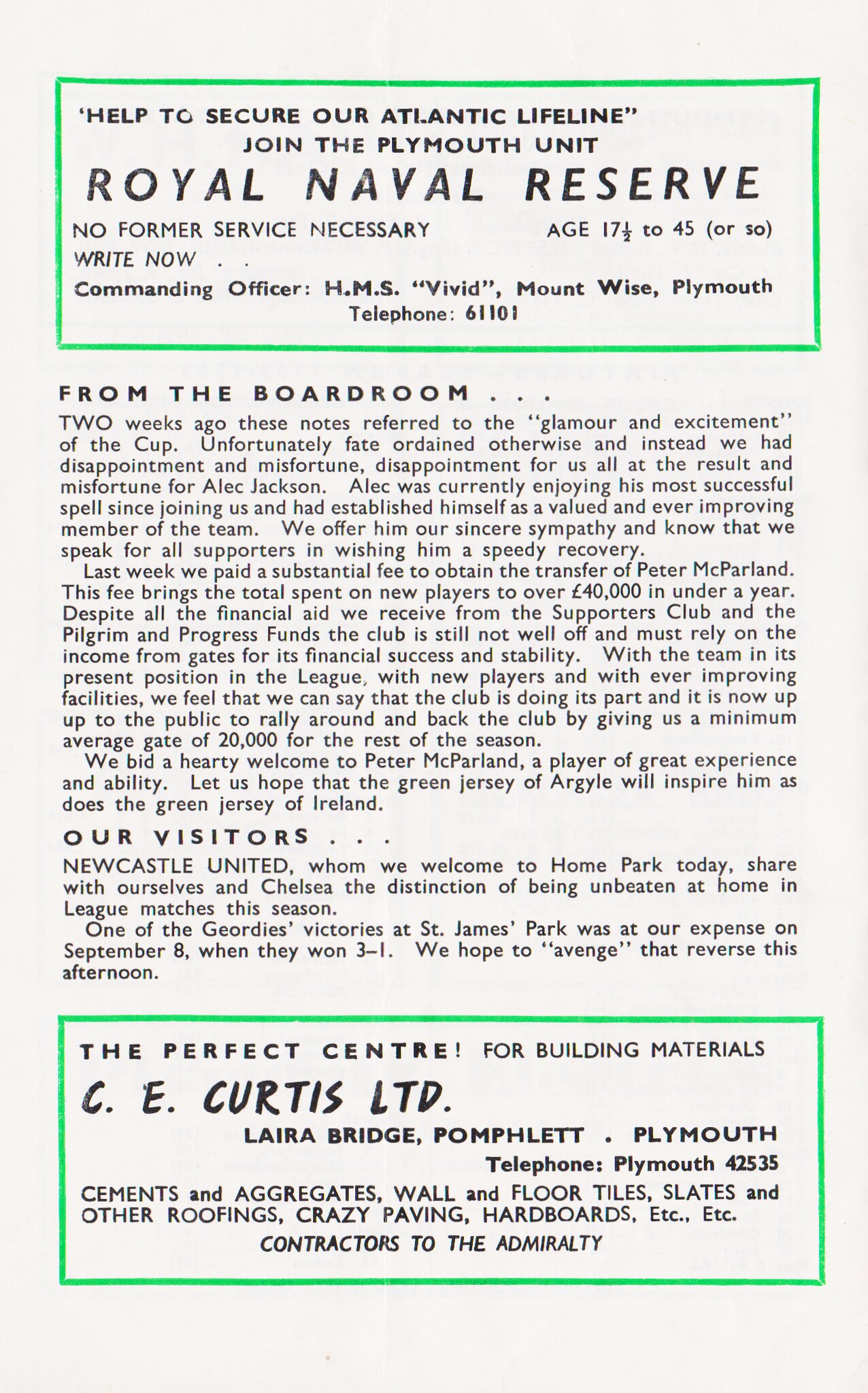This image showcases a black and white printed flyer with prominent ads, bordered by two thin green rectangles at the top and bottom. The top green-bordered banner features an advertisement in black text, urging viewers to "Help to secure our Atlantic lifeline. Join the Plymouth Unit, Royal Navy Reserve. No former service necessary, age 17 to 45," followed by contact information: "Commanding Officer HMS Vivid, Mount Wise, Plymouth. Telephone 61101." Below this, the text becomes difficult to read due to its small size but includes a section starting with "From the boardroom," discussing recent events related to a cup and mentioning a disappointment involving Alec Jackson. The flyer continues with several more paragraphs of text that are too small to decipher. At the bottom, another green-bordered panel advertises "The Perfect Center for Building Materials" by C.E. Curtis Limited located at Laira Bridge, Plymouth, offering products such as cement, aggregates, wall and floor tiles, slats and roofing materials, crazy paving, and hard boards, noting that they are contractors to the Admiralty.